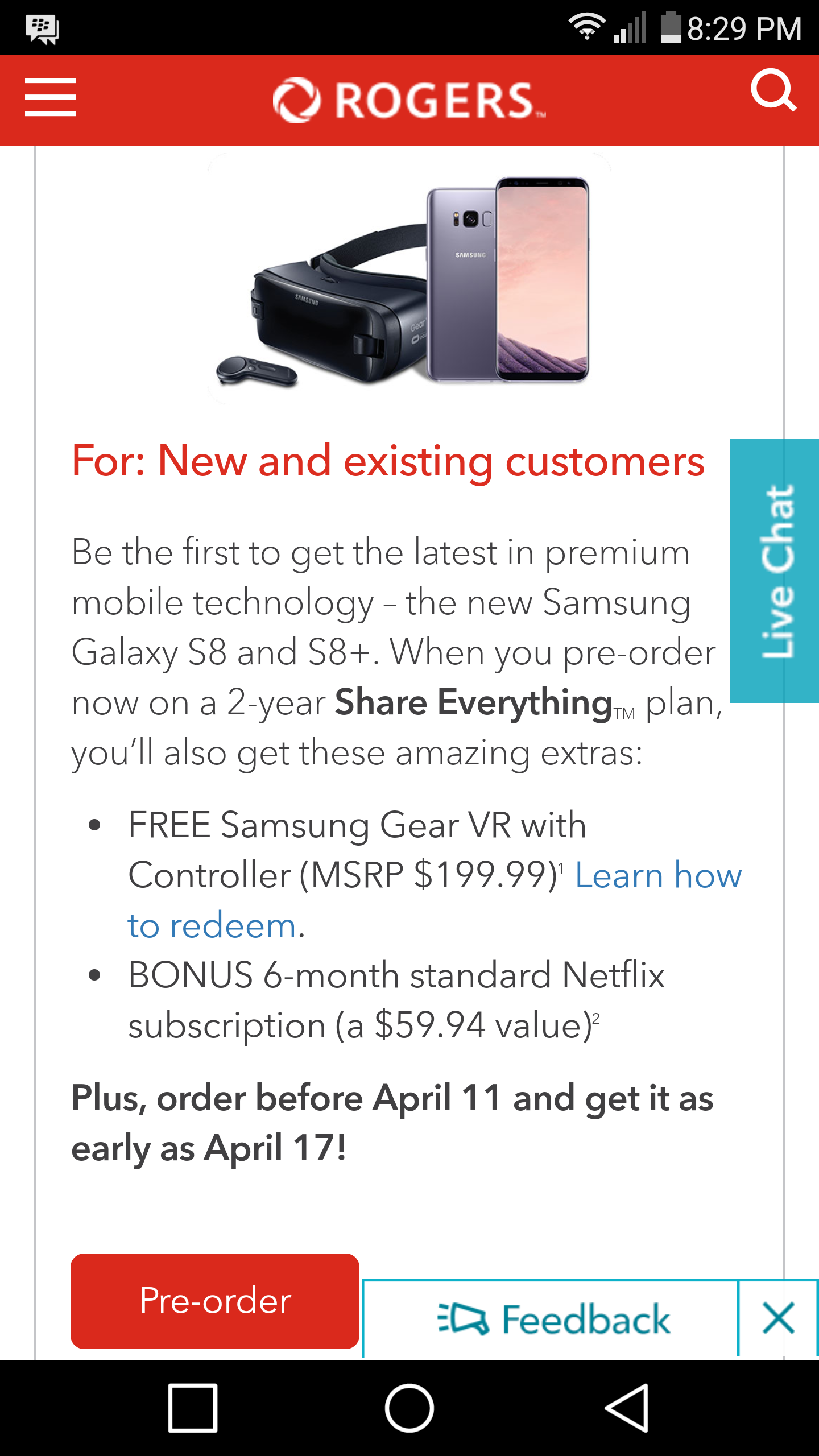A screenshot from a Rogers website shows the promotion of the new Samsung Galaxy S8 and S8+ smartphones. The main section features an image of the phone alongside a Samsung Gear VR headset. The text promotes an offer for both new and existing customers: "Be the first to get the latest in premium mobile technology, the new Samsung Galaxy S8 and S8+." Customers who pre-order on a two-year Share Everything plan will receive a free Samsung Gear VR with controller, valued at $199.99. Additionally, a six-month standard Netflix subscription, valued at $59.94, is included. A highlighted note mentions that orders placed before April 11th may be received as early as April 17th. Below this, there is a "Pre-order" button, as well as a "Give Feedback" button. A live chat option is available at the top of the webpage. 

At the very top of the screenshot, standard phone indicators are displayed, including Wi-Fi signal strength, cellular service signal, battery life, and the current time, 8:29 p.m. There are also icons for chat and a dropdown menu.